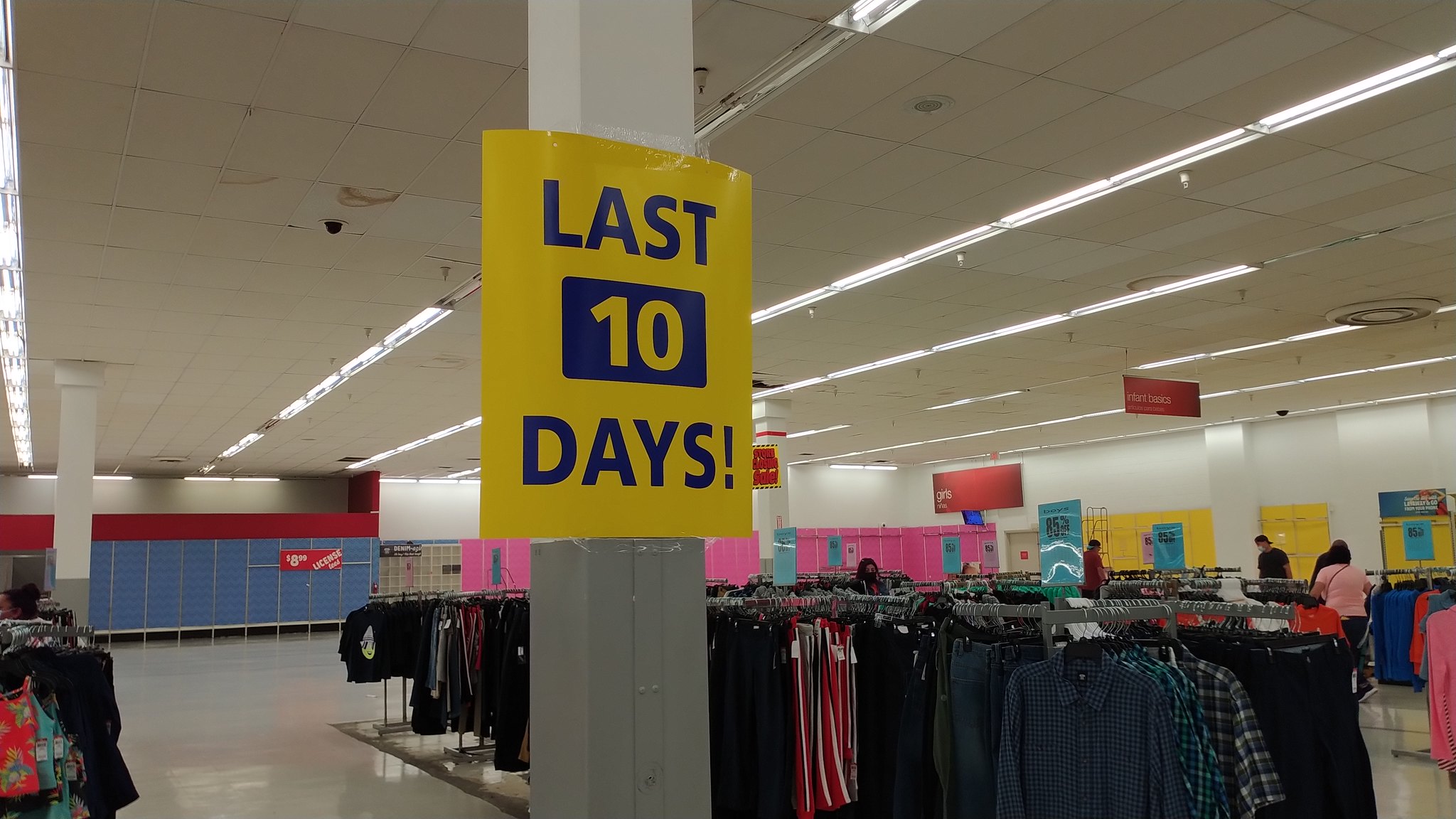This photograph showcases the interior of a largely empty clothing store. The upper two-thirds of the image is dominated by a white tiled ceiling, featuring six tracks of fluorescent tube lighting that span across the entire ceiling. In the forefront, a white and gray support beam stands prominently, adorned with a yellow sign. The sign, made of yellow paper with blue font, declares "Last 10 Days" with the number "10" enclosed in a blue box, matching the yellow background. The lower portion of the photo reveals several racks of clothing situated behind the beam, predominantly displaying men's apparel.